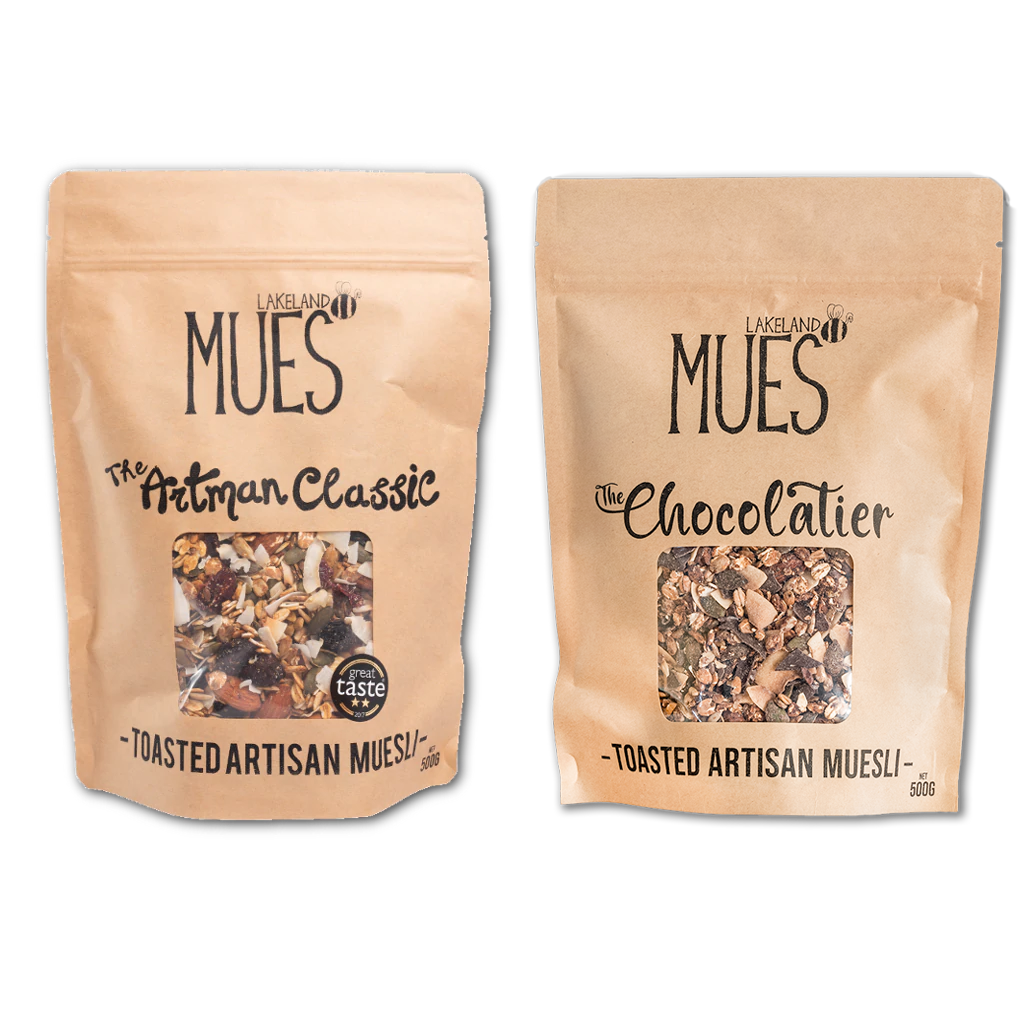This color photograph features two beige-brown packages of muesli on a white background. Each package is labeled "Lakeland Muse" with a black outline of a bumblebee next to the brand name. The left package is named "The Artman Classic" and the right one is called "The Chocolatier," both in black cursive font. A clear, plastic window on each package reveals the contents, which appear to be a mix of raisins, slivered almonds, seeds, nuts, and chocolate pieces. Below the window, the words "Toasted Artisan Muesli" are prominently displayed in black capital letters, with "500G" marked on the bottom right corner of each bag.